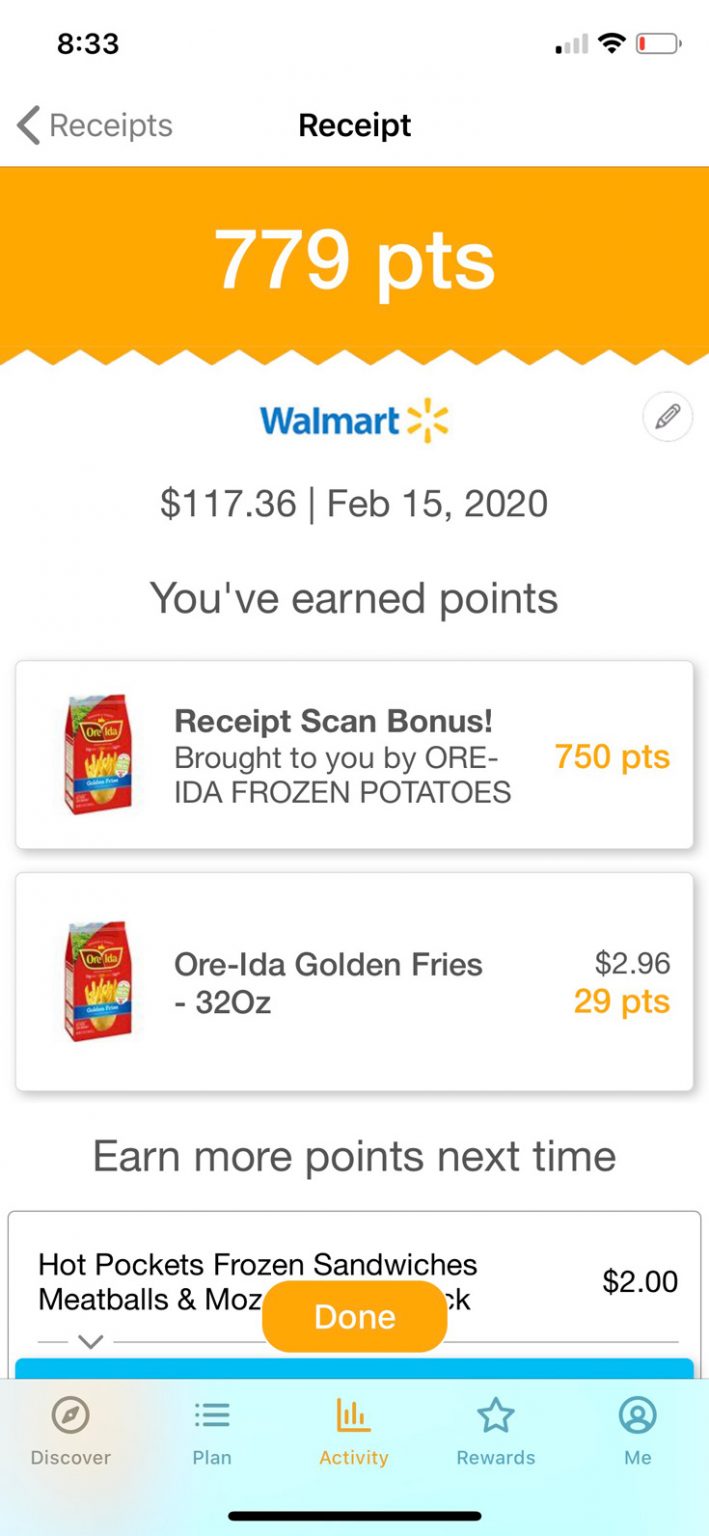On a stark white background, there is a detailed representation of a scanned receipt in gray tones. Dominating the top portion is an orange rectangle emblazoned with '779 points', signaling a reward system. Below this, the receipt prominently features the Walmart logo alongside the date 'February 15th, 2020'. The total amount spent is listed as $117.36. A message proudly states 'You've earned points' followed by a 'Receipt Scan Bonus' brought to you by Ore-Ida Frozen Potatoes, specifically for a purchase of 'Golden Fries (32 oz)' which earned 750 points and cost $2.96. 

Though some text is truncated, it also documents the purchase of Hot Pockets Frozen Sandwiches—likely the Meatballs and Mozzarella variety—priced at $2. A yellow oval with the word 'Done' in white suggests completion of input or scanning. Interspersed text encouraging users to earn more points next time hints at a loyalty or rewards program. The bottom of the image showcases navigation headers like 'Discover', 'Plan', 'Activity', and 'Rewards Me', while a black bar stretches across the bottom center, possibly indicating a navigation or status bar.